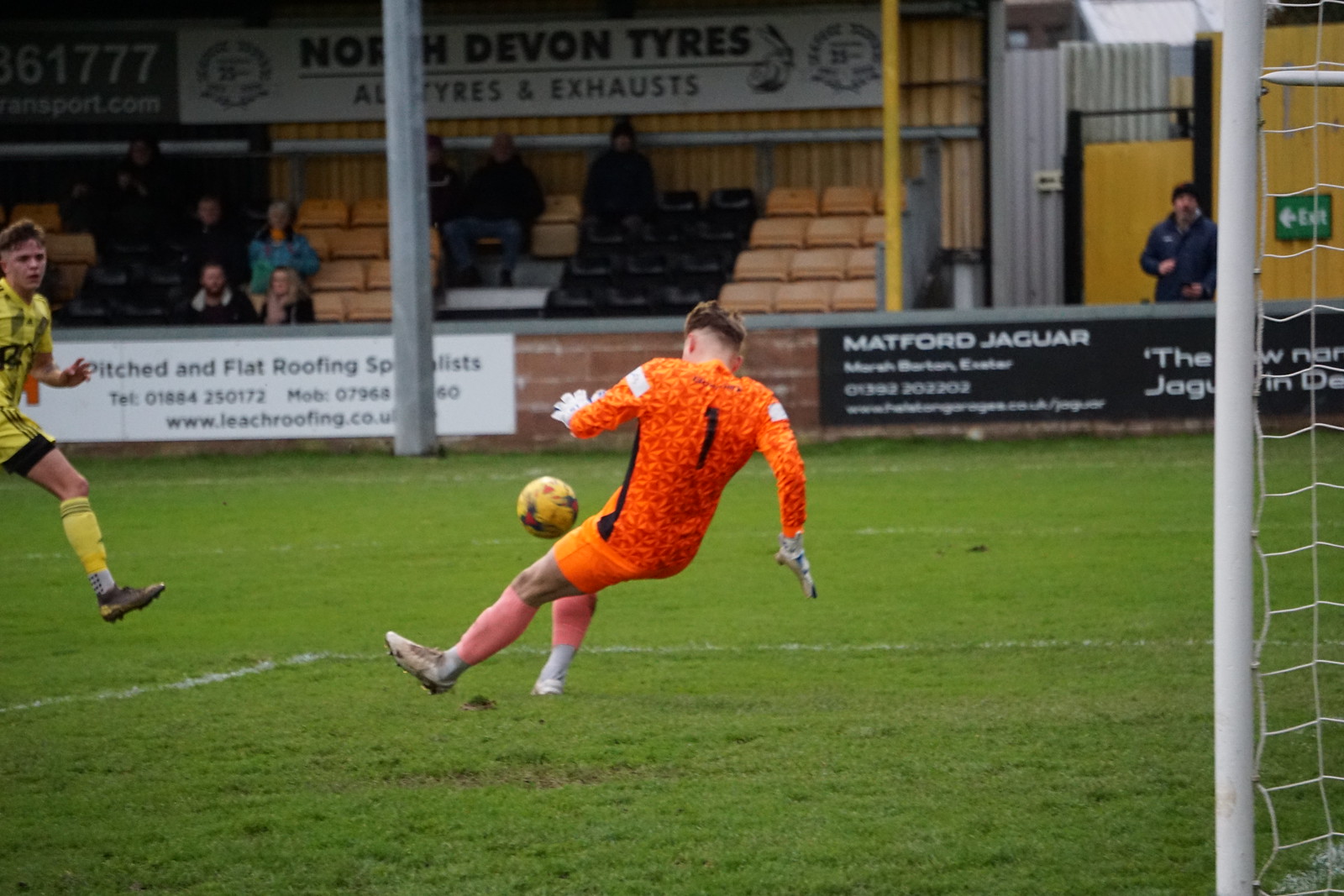The photograph captures a dynamic moment during a soccer game on a green field. The focal point is an athletic goalkeeper dressed in an orange uniform with white shoes and distinctive pink socks, diving to his right in a dramatic effort to catch a yellow soccer ball. The ball appears to have been shot by a player in yellow, barely visible on the left edge of the frame. The goalkeeper, positioned inside the penalty box, is either diving or leaning backward almost horizontally, with one foot still on the ground. To the right, part of the white goal net is visible. In the background, a red brick wall with gray capping and two sponsor signs, one white and one black, can be seen. Beyond the wall, there are raised bleachers with about ten spectators, underlining the organized setting of the game.